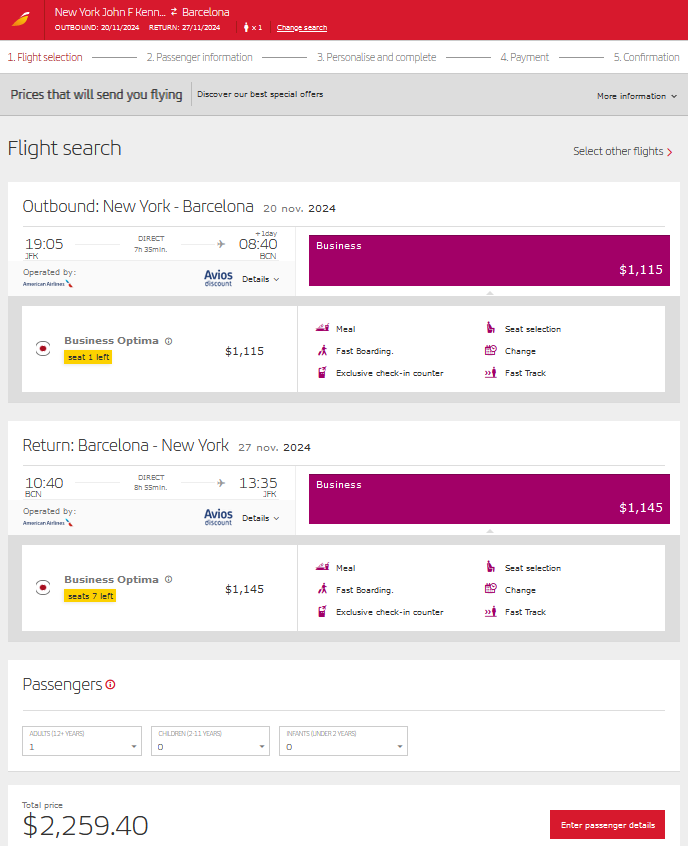The webpage displayed is a flight booking platform, showcasing detailed options for a trip from New York to Barcelona on November 20th, 2024. The outbound flight departs from JFK and is a direct route to Barcelona, lasting 7 hours and 35 minutes. This particular flight option is classified under "Business Optima" and includes amenities such as a meal, fast boarding, access to an exclusive check-in counter, seat selection, the ability to make changes, and fast track services. Currently, there is only one seat left for this flight, priced at $1,115.

The return flight from Barcelona to JFK departs at 10:40 AM and arrives at 13:35 PM, spanning a duration of 8 hours and 55 minutes. This return flight is also a direct route and falls under the same "Business Optima" class, offering identical amenities as the outbound flight. There are seven seats available, each priced at $1,145.

Additionally, the webpage features a section where passengers can select the number of adults, children, and infants traveling. Booking both the outbound and return flights results in a total cost of $2,259.40.